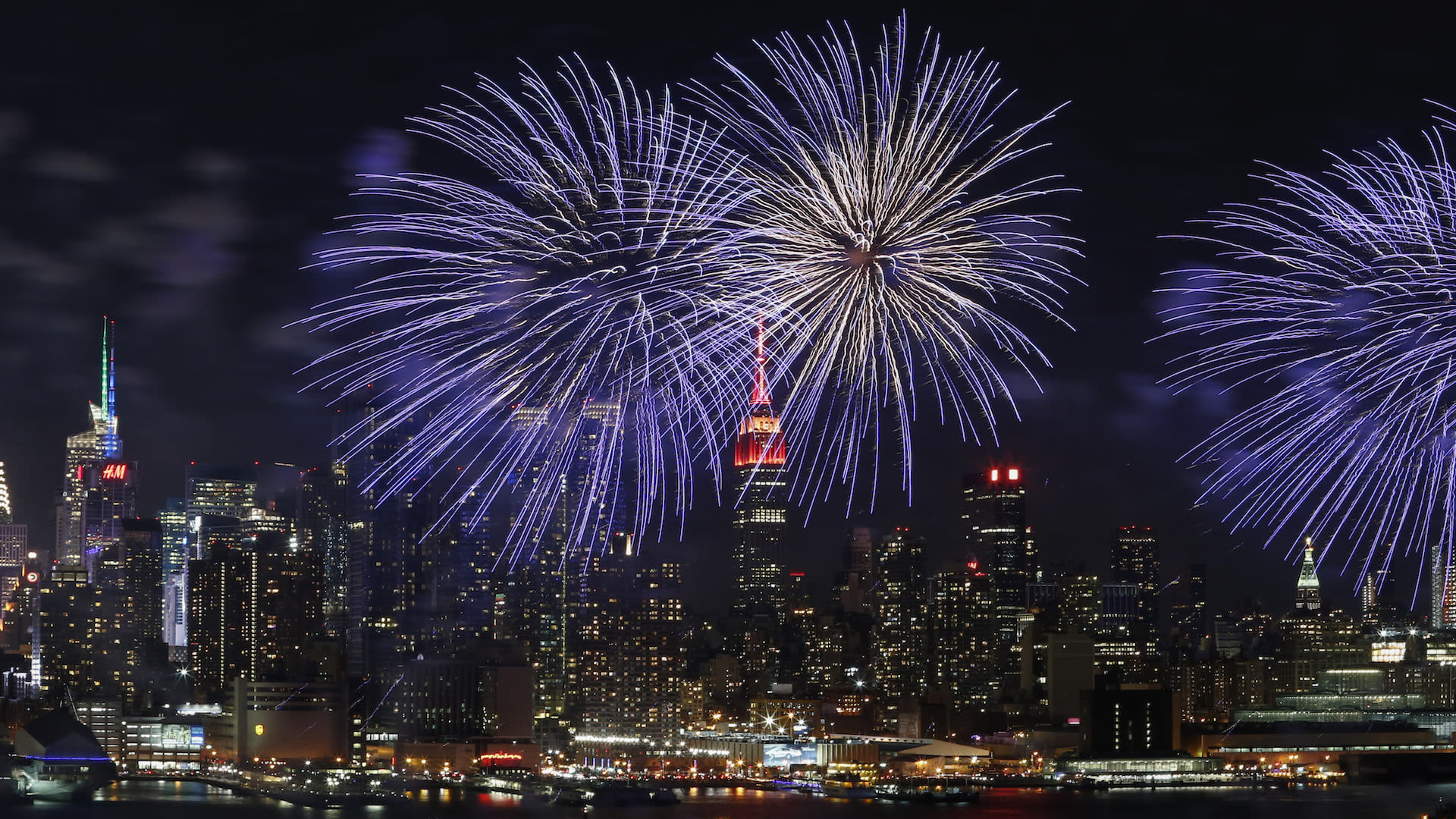The image is a landscape orientation color photograph capturing an enchanting nighttime view of the downtown New York City skyline, prominently featuring several towering buildings illuminated from within. The skyline stretches across the background, while the foreground reveals a piece of the Hudson River, reflecting the city's lights and showcasing several boats along the shoreline.

Above the cityscape, three grand explosions of fireworks dominate the top portion of the image, spanning from the middle left to the middle right. These fireworks bursts are primarily a light purple or lavender hue with lighter centers, casting vibrant streams of color across the night sky. The leftmost burst is slightly lower than the central one, while an additional cluster of fireworks embellishes the right side of the skyline.

The scene is framed by a solid black sky, emphasizing the vivid colors and intricate details of the lit windows in the buildings below, as well as the shimmering reflections in the water. This detailed photograph embodies a realistic, representational style, capturing the dynamic essence of a celebratory night in New York City, potentially from a video freeze-frame.